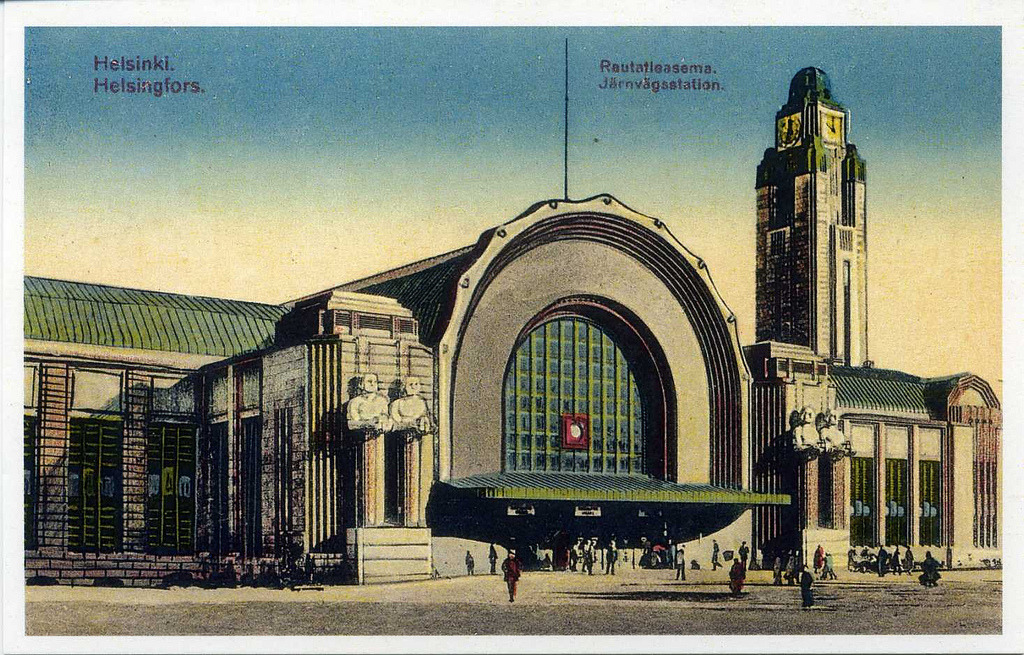This detailed drawing, evocative of a mid-20th-century postcard, depicts a grand stone building situated in Helsinki (referred to as Helsingfors in Swedish). Dominating the architecture is a large archway entrance, embellished with a glass window comprising many panes. Centrally positioned within the window is a small red object. Flanking the entrance are statues, representing human torsos and heads, set upon columns. Above the entrance, a roof extends outwards, casting a protective shadow.

In the background, a prominent clock tower rises, topped with a dome and displaying clocks on all four sides. The sky behind the building transitions from a dark blue at the top to a lighter white near the horizon. Adding to the historical charm, the building is depicted with intricate brickwork and large windows, while a group of people is captured entering and exiting the bustling structure. The image suggests the building might be a significant transportation hub or station, given its architectural grandeur and the flow of people. The text “Helsinki. Helsingfors.” is displayed in deep red in the upper left corner, reinforcing the postcard feel of the image.